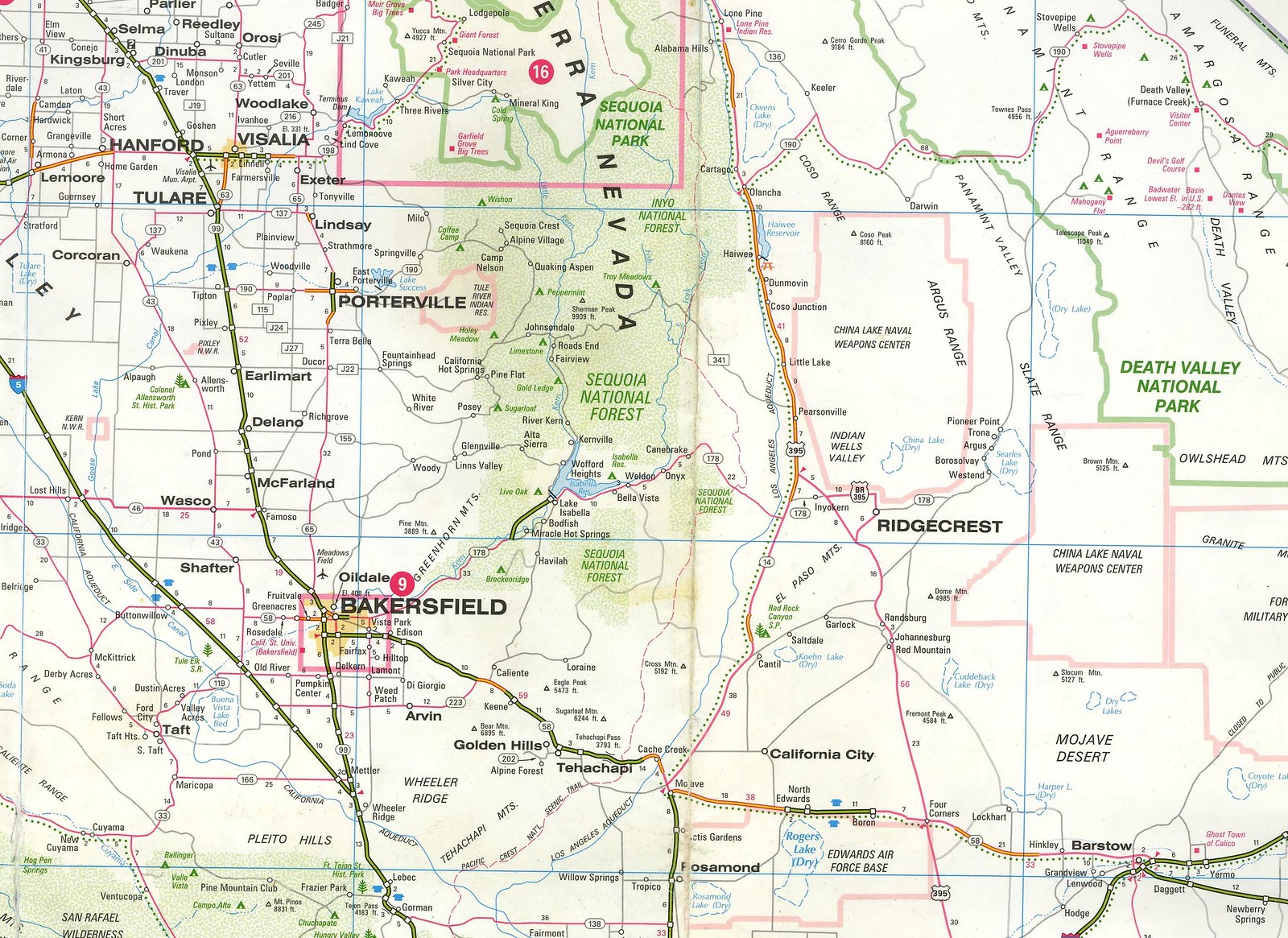The image depicts a segment of a detailed map set against a cream-colored background. The map highlights various cities and towns, with the size of the town names correlating to the population size—larger cities are marked with larger text. Green areas depict forests, while green lines trace the roads traversing the depicted region. The map specifically focuses on an area of California, prominently featuring Bakersfield and the Sequoia National Forest. Highways are clearly marked, and tiny triangular symbols represent campsites scattered across different locations. Parks and notable sightseeing areas are labeled in red text. Additionally, dotted lines follow certain roads, perhaps indicating routes or trails. Despite its detail, the map lacks a legend and a scale for measuring distances.